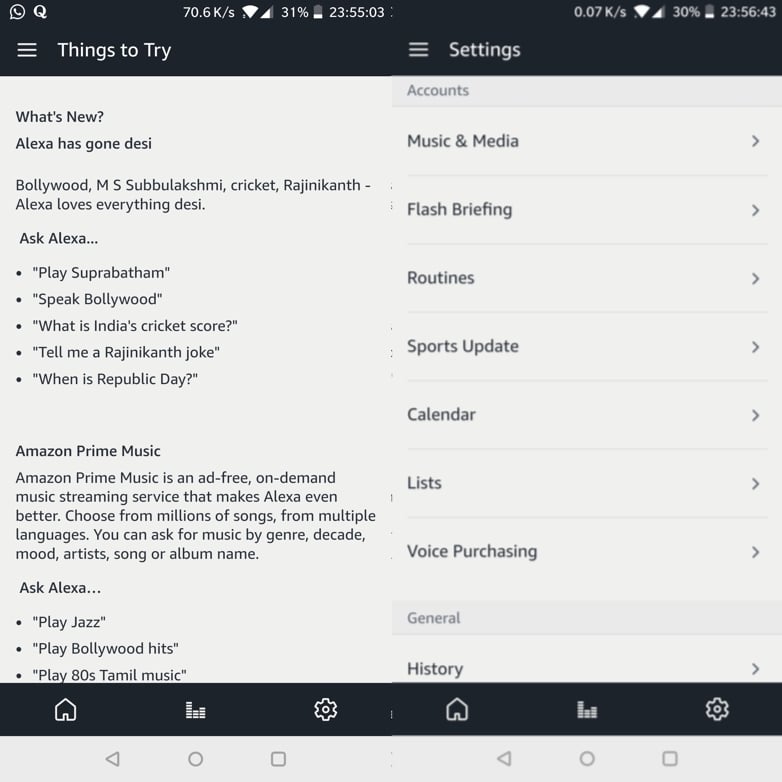The screenshot captures the interface of a mobile phone, displaying various features and settings associated with Alexa. At the top of the screen, the battery indicator shows a charge level of 31%, and the time is 23:55, which is just before midnight. Below this, there are two headers labeled "Things to Try" and "Settings," each accompanied by a hamburger menu for further options.

Under the "Things to Try" section, several suggested actions are listed:
- "Let's see what's new" prompts the user to explore recent updates.
- A humorous line states, "Alexa has gone dazzy. Uh-oh." followed by Alexa’s response, "Hmm, I don't know that."
- The user offers an apology with, "Yeah, sorry Alexa."
- The section continues with a topic suggestion of "Bollywood."
- Further suggestions encourage the user to ask Alexa about Amazon Prime Music with the prompt "Ask A-L-E-X-A."

In the "Settings" section, various customization options are visible, allowing the user to tailor their Alexa experience:
- Music and Media
- Flash Briefing
- Routines
- Sports Update
- Calendar
- Lists
- Voice Purchasing
- History

The caption concludes with a question to Alexa, "Is that good with you, Alexa?"

Overall, the screenshot provides a detailed look at the mobile interface for managing Alexa's features, highlighting specific prompts and settings for user interaction.